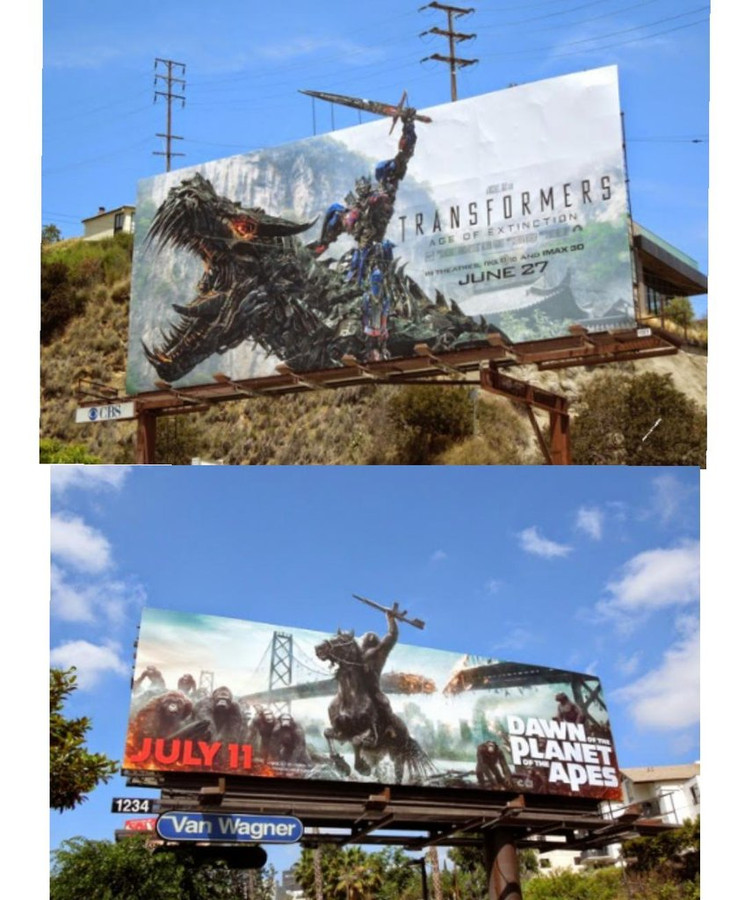The image features two vibrant, side-by-side, landscape-oriented photographs, each depicting an outdoor billboard advertising upcoming movies. 

The top billboard announces "Transformers: Age of Extinction," set to release on June 27th. Dominating the scene is a mechanical dragon, its head facing left. Beside it stands a large transformer, vividly detailed with red and blue hues, brandishing a sword in its left hand. The sword dramatically extends outwards at a 45-degree angle, piercing beyond the confines of the billboard's rectangular frame.

The lower billboard, set against a backdrop of a blue, daytime sky speckled with wispy white clouds along its edges, promotes "Dawn of the Planet of the Apes," slated for release on July 11th. This advertisement showcases an intense scene with apes and a partially bucking horse. Though slightly unclear due to image quality, an ape is discernible atop the horse, gripping a gun that points skyward beyond the billboard’s border. Behind them, a bridge looms in a state of fiery destruction, parts of it crumbling dramatically.

Both billboards employ dynamic, immersive elements that extend into the surrounding environment, bringing the advertised action to life.